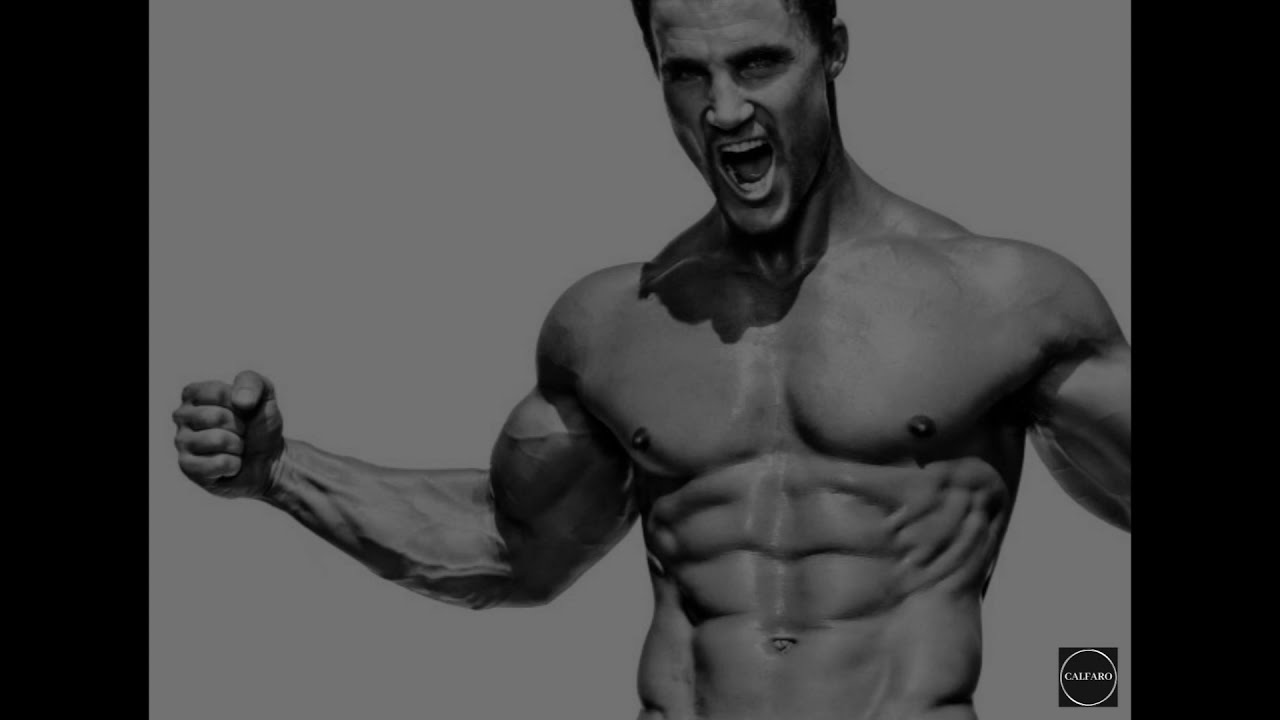This black and white advertisement features a highly muscular, shirtless man with short dark hair. The top of his head is slightly cropped out of frame, but his striking light eyes and dark eyebrows are visible. He stands against a grayish white wall, flanked by two black vertical banners on either side. The man is depicted in a powerful, almost bear-hug pose, with his mouth wide open as if screaming. His physique is accentuated, showcasing his bulging biceps, forearms with visible veins, deltoids, triceps, pectoral muscles, and a prominent six-pack that melds seamlessly into his ribcage. His nipples are erect, and his belly button is visible. At the bottom right corner of the image, there is a logo featuring the text "Calfaro" written in white within a black box.